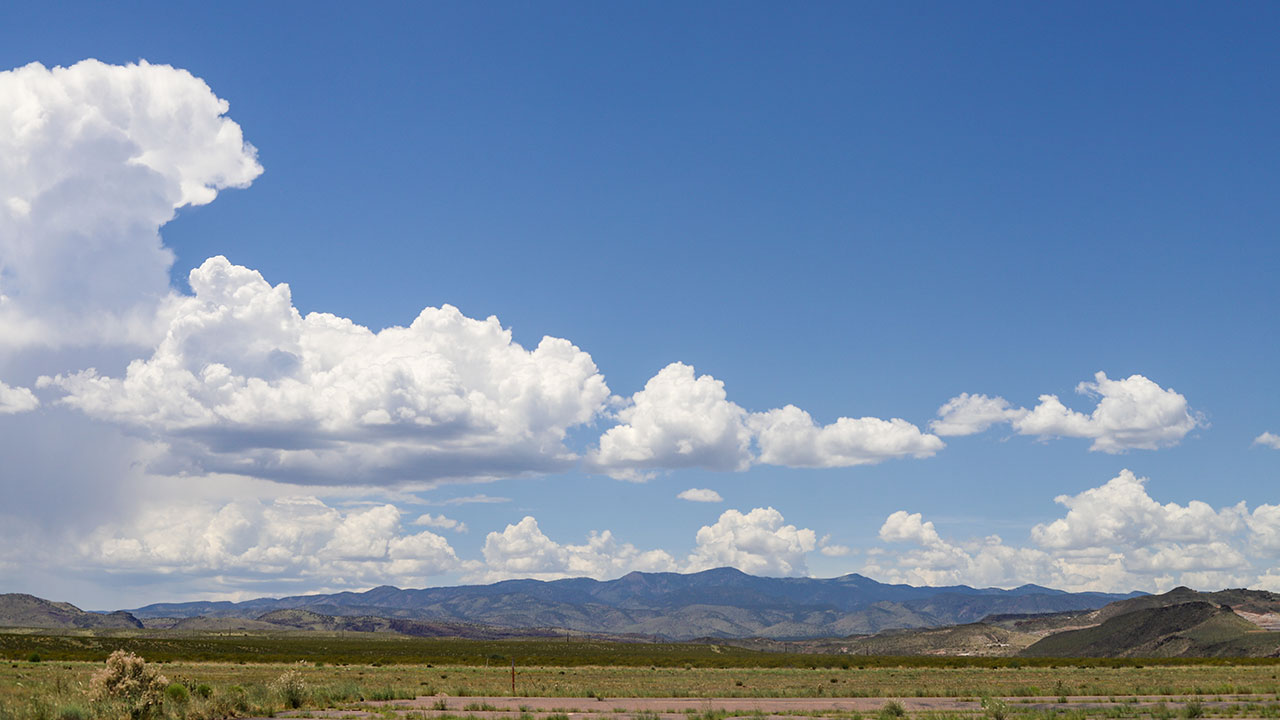The photograph captures a stunning landscape featuring a flat, brushy field with patches of bare soil, transitioning into more lush greenery as the distance increases. In the foreground, there is a road flanked by grass that becomes progressively darker green. Beyond the grassy area, rolling hills rise up, leading to small mountains in the far distance, which have a dark blue hue. The sky occupies approximately 75% of the image, showcasing a vibrant blue expanse dotted with numerous fluffy white clouds, with some gray streaks primarily on the left side. The clouds predominantly gather in the lower portion of the sky, emphasizing the expansive, open feel of the scene. The overall setting appears reminiscent of a Colorado prairie field during summertime, characterized by its vivid colors and lack of snow, underscoring the serene beauty of the landscape.